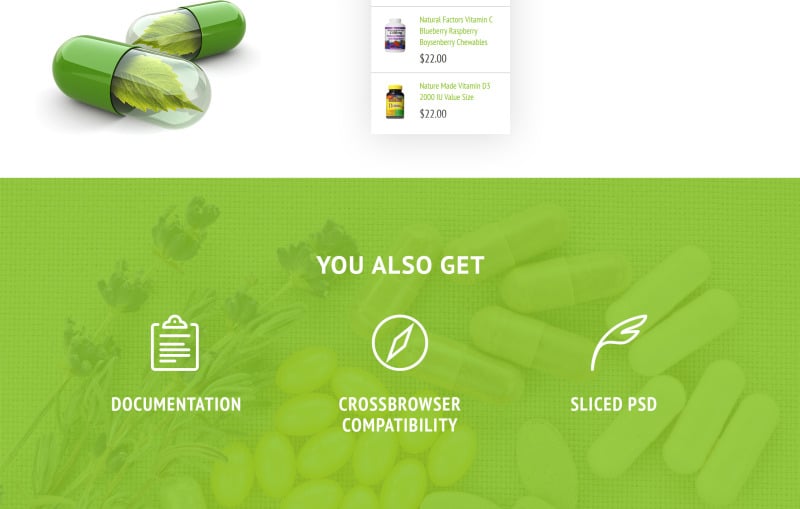Zoomed in on the image, the viewer can observe a detailed layout. Front and center is a large, green rectangular display featuring shadows of some pills. To the left of this display, delicate branches of flowers are visible. The display itself provides text information, stating that you receive documentation, cross-browser compatibility, and sliced PSD files.

Prominently above the text, two capsule pills are displayed. Each pill is half green and half clear, with a small green leaf encapsulated inside. Below this section, two small boxes feature images of pill bottles.

The first box showcases a bottle labeled "Natural Factors, Vitamin C." Priced at $22, these chewable vitamins come in flavors of blueberry, raspberry, and boysenberry. The second box features a bottle of "Nature Made, Vitamin D3 2000 IU," designated as a value size. This product is also available for $22.